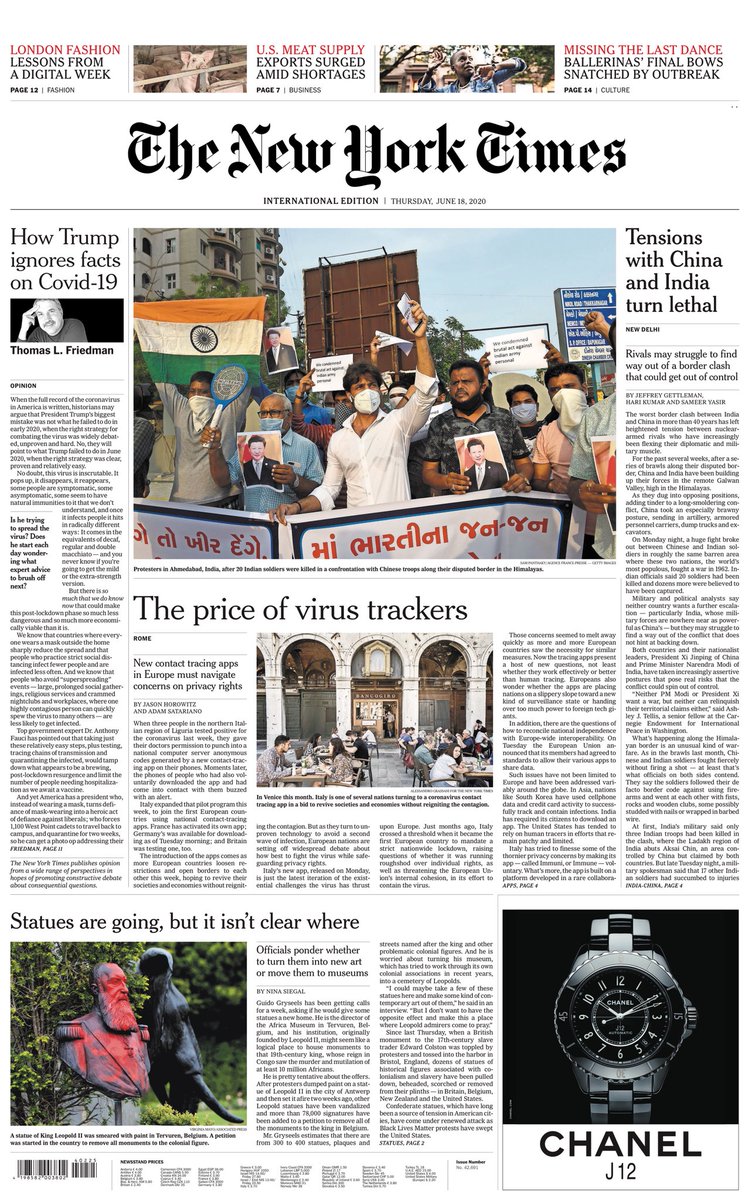Today’s front page of the International Edition of The New York Times, dated June 18, 2020, features a comprehensive array of articles offering a snapshot of global and national issues. 

At the top, three highlighted articles preview what's inside: 
- "London Fashion" on page 12, teasing insights from a digital fashion week.
- "U.S. Meat Supply," discussing the surge in exports amid domestic shortages.
- "Missing the Last Dance," focusing on challenges faced by ballerinas.

The page is divided into three main columns. On the left, an opinion piece by Thomas L. Friedman titled "Trump's Annoying Facts on COVID" delves into the handling of the pandemic, accompanied by a boxed quote highlighting a key argument from the column.

The central column features an image capturing a tense moment near the Himalayas, with local citizens holding signs, their national flag, and an image of their president. The article, "The Price of Virus Trackers," addresses the societal costs of surveillance measures introduced to curb the pandemic.

On the right, the lead story, "Tensions with China and India Turn Lethal," covers the escalating border conflicts and explores the difficulties these rivals face in resolving their disputes peacefully.

Below these main stories, two additional articles are presented:
- An in-depth piece on virus trackers and their implications.
- An exploration of the growing debates over statues, both pointing towards the shifting societal attitudes.

To the far right, an opulent advertisement for the Chanel J-12 watch adds a touch of luxury to the page.

Overall, the front page blends urgent news with diverse topics ranging from international tensions to cultural shifts, offering readers a detailed portrayal of current events.